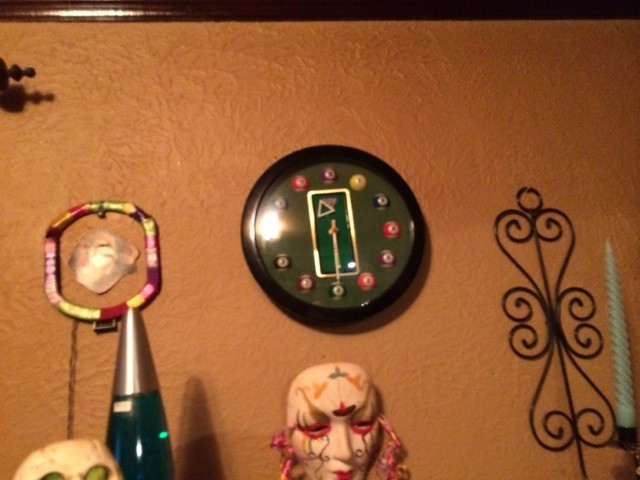This vibrant image showcases a creatively decorated wall bathed in an orangish, burnt sienna hue with a brown border running across the top. The focal point is a distinctive billiards-themed clock at the center. Encased in black, the clock's face features a green felt background, resembling a pool table. The numbers on the clock are represented by billiard balls, arranged in traditional clockwise order. The clock's hands are designed as pool sticks, pointing towards the 6, and the clock's face includes a small, triangular pool ball rack between the 12 and 11 positions, emphasizing its unique theme. Below and around this striking clock, the wall is adorned with an array of eclectic items. Directly beneath the clock is a Venetian or Mardi Gras-style clown mask, featuring a white face with pink around the eyes, gold detailing, and streamers. To the bottom left of the mask, a dark blue, partially off-screen lava lamp with a silver cap is positioned. Adjacent to this is another mask with green eyes peeking just above the frame. On the right side of the clock, a long, spiraled candle stands near a black steel wall sconce with leaf designs and a ribbed blue votive candle. Additionally, a small, colorful rectangular decoration with a monkey mask motif and various hues of orange, yellow, green, pink, and purple adds to the eclectic mix. This decorative setup, while visually busy, vividly captures a blend of personal interests and memorabilia.